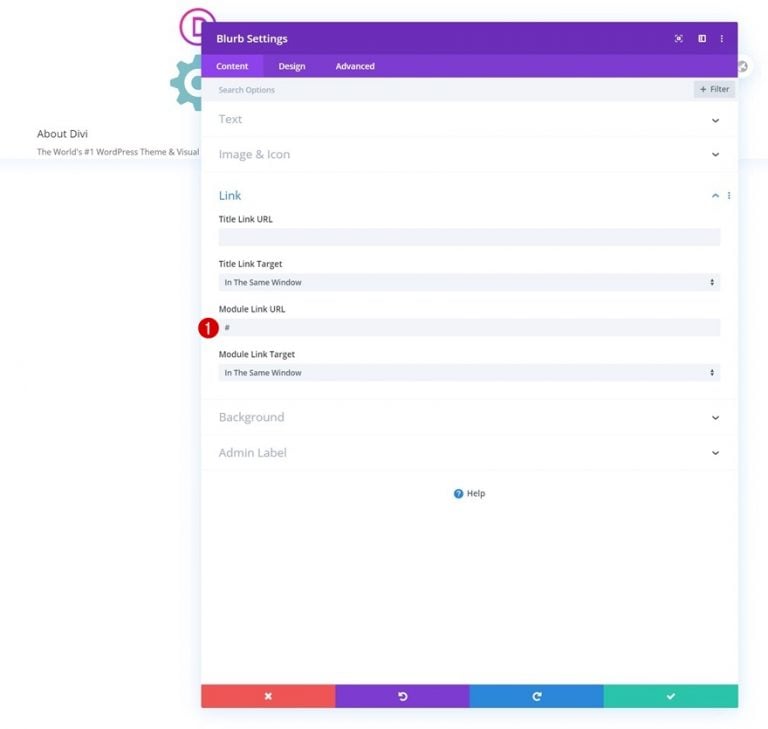Certainly! Here's an improved and detailed caption for the described image:

---

The image appears to be a screenshot of a computer screen displaying part of a WordPress interface using the Divi theme. The background screen is predominantly white with a central purple circle and a gear icon, suggesting settings or customization. Text on the background reads, "About Divi, the world's number one WordPress."

Covering the upper central part of the screen, there is a pop-up rectangle with a purple border labeled "Blurb Settings" in the upper left corner. This pop-up features three tabs: "Content," "Design," and "Advanced," with the "Content" tab currently selected.

Within the "Content" tab, the interface displays various options:
- A white search bar at the top labeled "Search Options."
- A section titled "Text" with options for "Image & Icon."
- A "Link" section with subheadings including:
  - "Title Link URL" accompanied by a gray input bar for entering a URL.
  - "Title Link Target" featuring a dropdown menu currently set to "In the Same Window."
  - "Module Link URL" with a corresponding input bar.
  - "Module Link Target" set by default to "In the Same Window."

Below these sections, there is a larger white area, and on the left side, two sections labeled "Background" and "Admin Label." In the lower center of the pop-up is a "Help" option.

At the bottom of the pop-up, there are four action buttons:
- A red button with an "X" icon, likely for closing or canceling.
- A purple button with a refresh icon.
- A blue button with a forward refresh icon.
- A green button with a checkmark, presumably for saving changes.

---

This detailed caption provides a clear and descriptive overview of the screenshot and its elements.